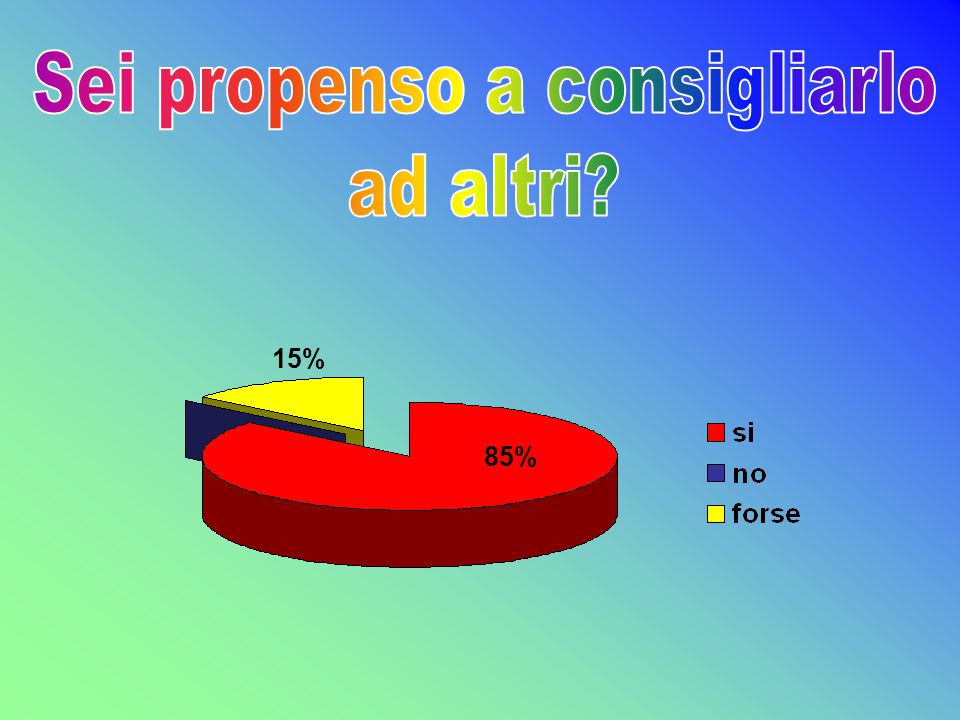The image features a colorful pie chart set against a gradient background that transitions from light green in the lower left to light blue and then dark blue in the upper right. At the top of the image, bold, rainbow-colored text in a Latin-based language—possibly Spanish or Italian—reads, "Sei propenso a consigliarlo ad altri?" with the initial letters of each word changing colors from red to purple. 

Centered prominently in the image is the pie chart, divided into three segments. The largest segment is red, representing 85% with the label "Sì" (yes). A very slim dark blue segment represents "No" without a specified percentage. The third and final segment is yellow, representing 15% with the label "Forse" (maybe). To the right of the pie chart, a legend clarifies the color coding: red for "Sí," dark blue for "No," and yellow for "Forse." The layout suggests a research setting with its clean design and apparent emphasis on survey results.